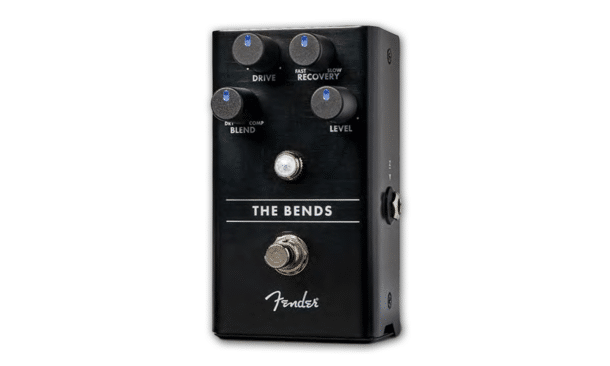This image features a rectangular, black guitar pedal made by Fender. The pedal, identified as "The Bends," is prominently labeled between two horizontal lines in the center. At the top, there are four knobs arranged in a rectangular configuration. The knobs, marked with blue arrows, are labeled "Blend," "Drive," "Recovery," and "Level," allowing users to adjust various sound settings. Just below these knobs is a small, white LED light, possibly indicating the pedal's operational status. Further down, a large silver button is present, likely serving as the activation switch for the pedal. At the bottom, the iconic Fender logo, written in white brush script, signifies the brand. Additionally, an auxiliary cord port is visible on the side of the pedal, indicating connectivity options.